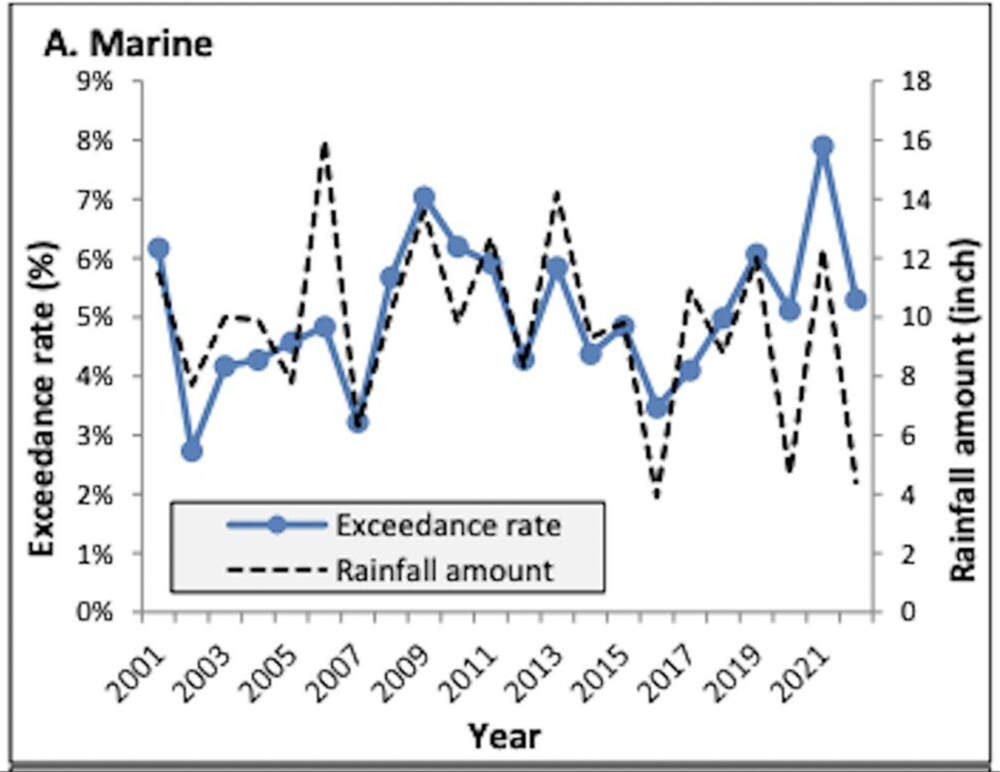This image features a detailed scientific graph titled "A, Marine," located in the top left-hand corner. The graph maps data from the years 2001 to 2021, displayed on the y-axis in intervals of two years. The left x-axis signifies the exceedance rate in percentage, ranging from 0% to 9%, while the right x-axis indicates the rainfall amount measured in inches, scaling from 0 to 18 inches in increments of two. Two distinct lines represent the key metrics: a solid blue line with blue dots for the exceedance rate, and a black dashed line for the rainfall amount. Notably, the highest rainfall amount was recorded in 2005, whereas the lowest was in 2021. Conversely, the exceedance rate peaked in 2021. The lines appear to be fluctuating independently across the graph, against a white background.